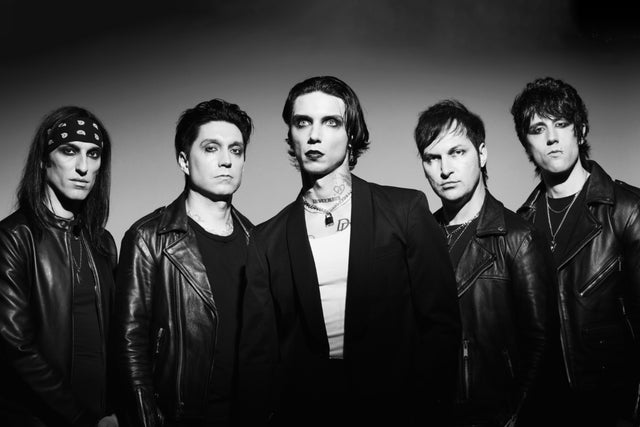This black and white photograph captures an emo rock band consisting of five men standing against a gradient background that transitions from dark gray to lighter gray. The band members are all dressed predominantly in black, with four of them wearing black leather jackets and the frontman in a black suit jacket over a white t-shirt, showcasing a padlock necklace. 

Starting from the left, the first man sports shoulder-length black hair, accentuated by black eye shadow and a black bandana with white spots. The second man has shorter, slicked-back black hair, and just stares stoically at the camera. In the center stands the frontman, distinguished by his heavier makeup that includes eyeliner and black lipstick, and mid-length black hair. To his left, the fourth member, also in a leather jacket, exhibits a disinterested gaze and has his black hair styled to the side. Finally, the man on the far right, with his black hair falling into his face and a slightly pouty expression, wears a pendant necklace.

Their collective expressions range from glowering to indifferent, encapsulating the quintessential moody aesthetic of an emo rock band.